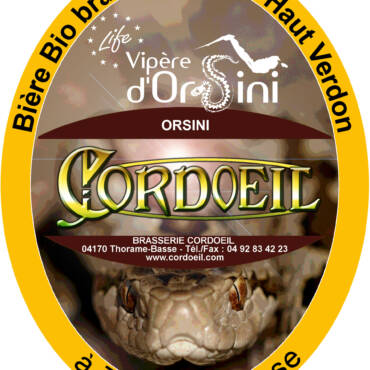The image is a detailed close-up of a product or logo against a white background, dominated by a vertically oriented, oval-shaped design that's partially cropped at the top and bottom. The oval is primarily yellow and divided into two sections. At the top left and right, thin black text spells "Be'er Bio," partially cut off at the top right corner by the phrase "Hout Verden."

Centrally within the oval, the word "life" is written in a white, almost cursive font, surrounded by a decorative circle of stars. Below this, in white text, it reads "Vipeer Doricini" (or “Vipeer Dorini”). Directly beneath this text, within a dark brown, oval bun-like shape, the word "Orcini" is written in white font. Further down, in a medieval, golden font featuring a large initial "C," the words "Cordo El" are presented.

At the very bottom, another brown bun-like shape contains the words "Brazier Corridor," along with what appears to be an address, telephone number, and website URL: "www.cordovel.com." Adjacent to this, the image features the head of a viper or snake, facing forward with light brown scales, black markings, golden eyes, and vertical black slit pupils, creating a striking focal point.